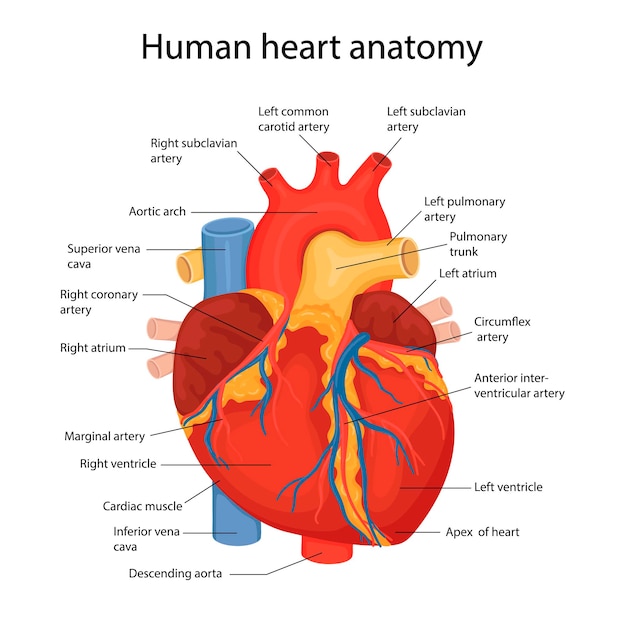This detailed illustration of the human heart, akin to those found in high school biology textbooks, is titled "Human Heart Anatomy" at the top and set against a white background. The heart itself is vividly colored, with red representing the main body, blue indicating veins and certain valves, and a yellowish tint highlighting other components. Each anatomical part of the heart is carefully labeled with lines connecting the labels to their corresponding locations. The labeled parts include the Descending Aorta, Inferior Vena Cava, Cardiac Muscle, Right Ventricle, Marginal Artery, Right Atrium, Right Coronary Artery, Superior Vena Cava, Aortic Arch, Right Subclavian Artery, Left Common Carotid Artery, Left Subclavian Artery, Left Pulmonary Artery, Pulmonary Trunk, Left Atrium, Circumflex Artery, Anterior Interventricular Artery, Left Ventricle, and Apex of Heart. This comprehensive depiction allows for an in-depth understanding of the heart's structure and function.